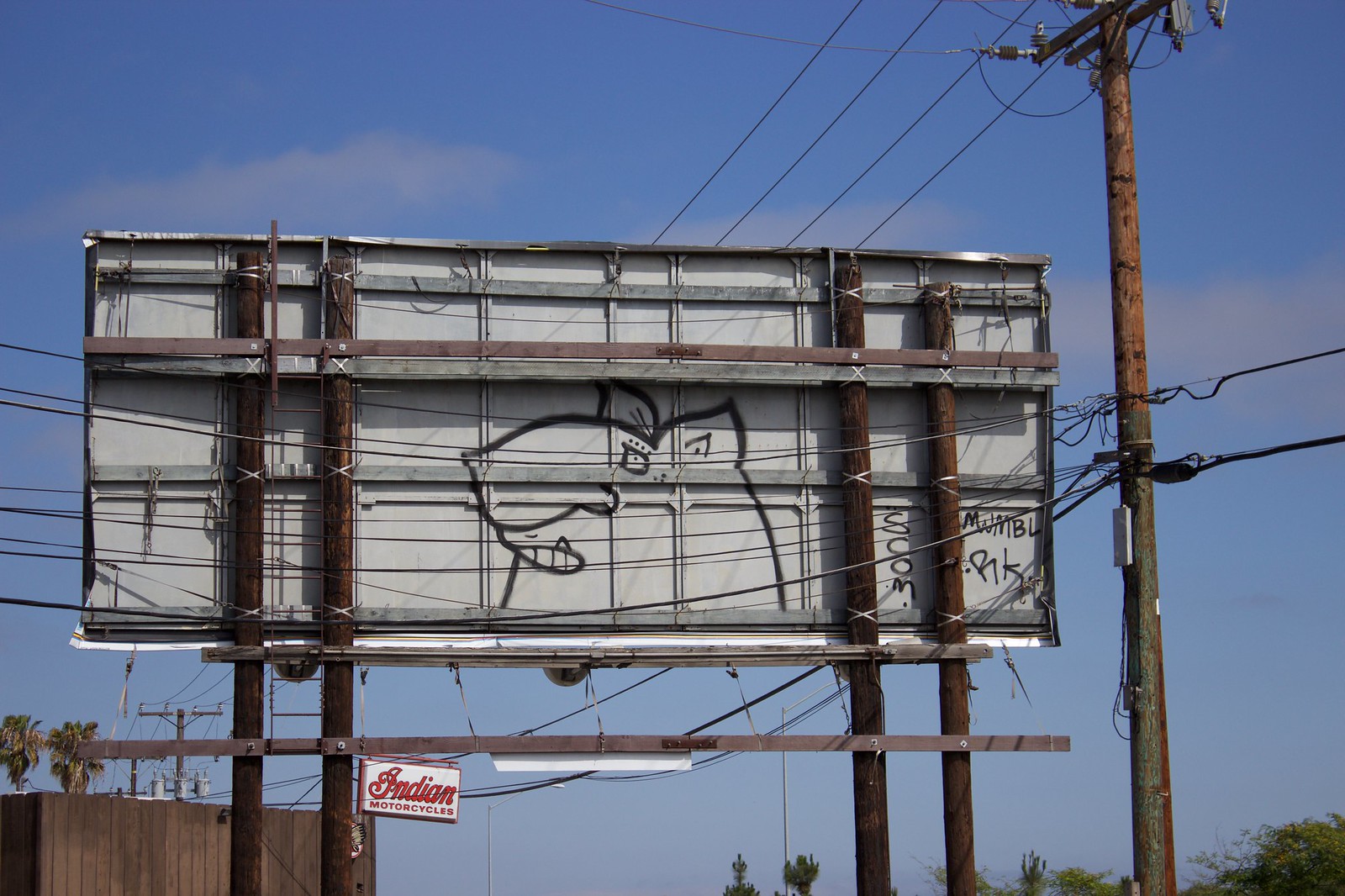In this image, we see the rear view of a large billboard, similar to those typically found along highways or city streets. The structure is supported by a combination of metal bars running horizontally and wooden poles positioned vertically. Numerous wires stretch across the back of the billboard, connecting to a nearby electric pole, highlighting the infrastructure's complexity. Notably, the back frame bears graffiti illustrating the head of a large, robust rat, adding an element of urban art. Affixed to the lower section of the horizontal bars is a sign that reads "Indian Motorcycles" in bold red letters against a clean white background. In the bottom left corner, a wooden fence is partially visible, and behind it, a couple of distant trees can be seen, providing a hint of the natural surroundings. The sky above is a serene blue, adorned with light, scattered clouds, suggesting a calm and pleasant day.